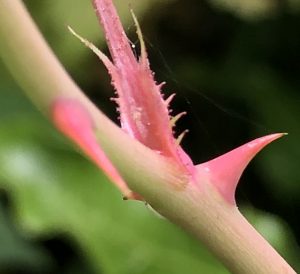This extreme close-up image captures the intricacies of a plant's stem, which runs diagonally from the upper left to the bottom right corner of the frame. The stem starts off with a pale peach tone that transitions into a whitish or off-white color as it progresses. Emerging from the stem are vibrant pink thorns, noticeably sharp and glossy, adding striking contrast. About two-thirds of the way down the stem, a prominent pink thorn juts out, while a spiky, pink offshoot resembling a new growth or flower also emerges near it. The pink parts of the plant appear wet and glossy, enhancing their vividness. In the blurred background, green foliage adds a lush, natural setting that draws attention to the detailed focus on the plant's stem and its intriguing textural elements.